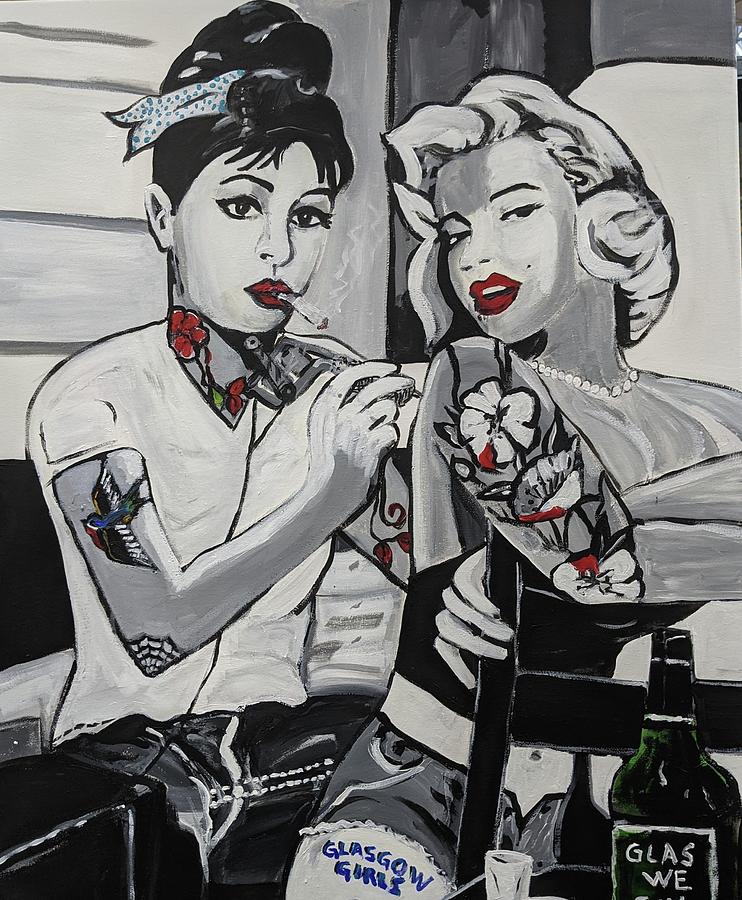The painting depicts two Caucasian women with light-colored skin, sitting next to each other. One woman, resembling Audrey Hepburn, sports a brunette updo adorned with a blue ribbon and has a cigarette in her mouth. She is decorated with neck and traditional old-school arm tattoos, holding a tattoo gun as she tattoos the other woman. The other woman, styled like Marilyn Monroe, has white-blonde hair and is adorned with bright ruby red lipstick. She wears a midriff-exposed tank top and short shorts, revealing a half-sleeve of floral tattoos on her upper arm. The phrase "Glasgow Girls" is visible over her leg. The painting is primarily in black, white, gray, blue, and red tones. A bottle of liquor and a shot glass sit in front of them, adding to the pin-up style vibe of the image. Additionally, both women's arms are rendered in a grayish tone that contrasts with their lighter-complexioned faces.